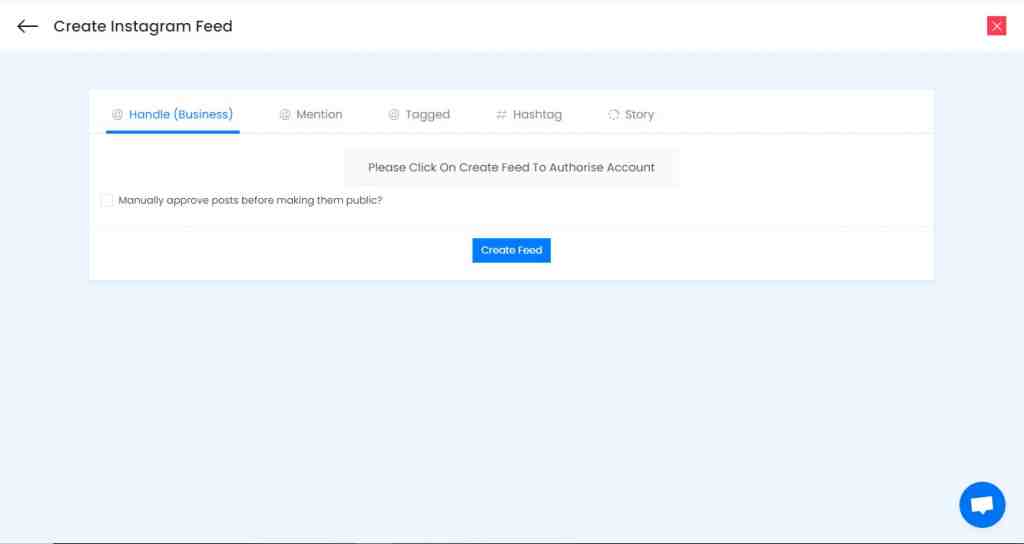The image primarily features a digital interface for managing an Instagram feed. In the top-left corner, there is black text that reads "Create Instagram Feed". Just to the left of this text, there is a prominent button.

The main section of the interface is dominated by a text box with a white background. Surrounding this central text box, the background is a light blue color. Within the text box, there are five tabs located at the top: "Handle Business", "Mention", "Text", "Hashtag", and "Store". All these tabs are written in gray, except for "Handle Business", which is highlighted in blue to indicate it is the currently selected tab. A blue line below the "Handle Business" tab further signifies its selection.

Centered within the text box is a message instructing users to "Please click on create feed to authorize account". Below this message, in the bottom-left corner, there is an unchecked checkbox labeled "Manually approve post before making them public".

In the bottom-center of the text box, there is a blue button with white text that says "Create Feed". 

For additional navigation, there is a red close button situated in the top-right corner of the interface. In the bottom-right corner, there is a chat icon colored blue with a white speech bubble inside it, indicating a conversation button for user support.